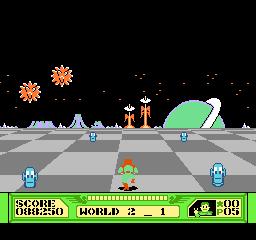This still image captures the essence of an old-school Arcade-style computer game set in the vastness of space. The top portion of the image is a solid black void, hinting at the boundlessness of the cosmos. Below, a wide band representing the in-game sky is also black but dotted with white stars, evoking a stellar backdrop. Within this starry expanse are two vibrant orange, sunburst-like shapes that resemble either dazzling fireworks or twin suns, adding a scintillating touch to the scene.

On the horizon line, grey pixelated mountains rise, creating a stark, otherworldly landscape. Standing prominently against these peaks are two orange humanoid figures, each with oval-shaped heads crowned with antennas, suggesting some form of alien life. Floating slightly above these figures, a green spherical object—possibly a planet—boasts a white ring tilted at a 45-degree angle, adding to the game's interstellar theme.

In the foreground, a dark and light grey checkered pattern covers the ground, lending depth and texture to the terrain. Among this checkered field are four small blue characters, each with expressive eyes that seem to peer into the distance. Centrally located is a unique character bearing both green and orange colors, standing as perhaps the protagonist or a significant figure in the game.

The bottom of the image features a green status band displaying the player's score and indicating that they are in "World 2." On the far right of this status bar, a drawing of a mysterious creature adds a final layer of intrigue and anticipation, hinting at the adventures that lie ahead in this captivating arcade universe.